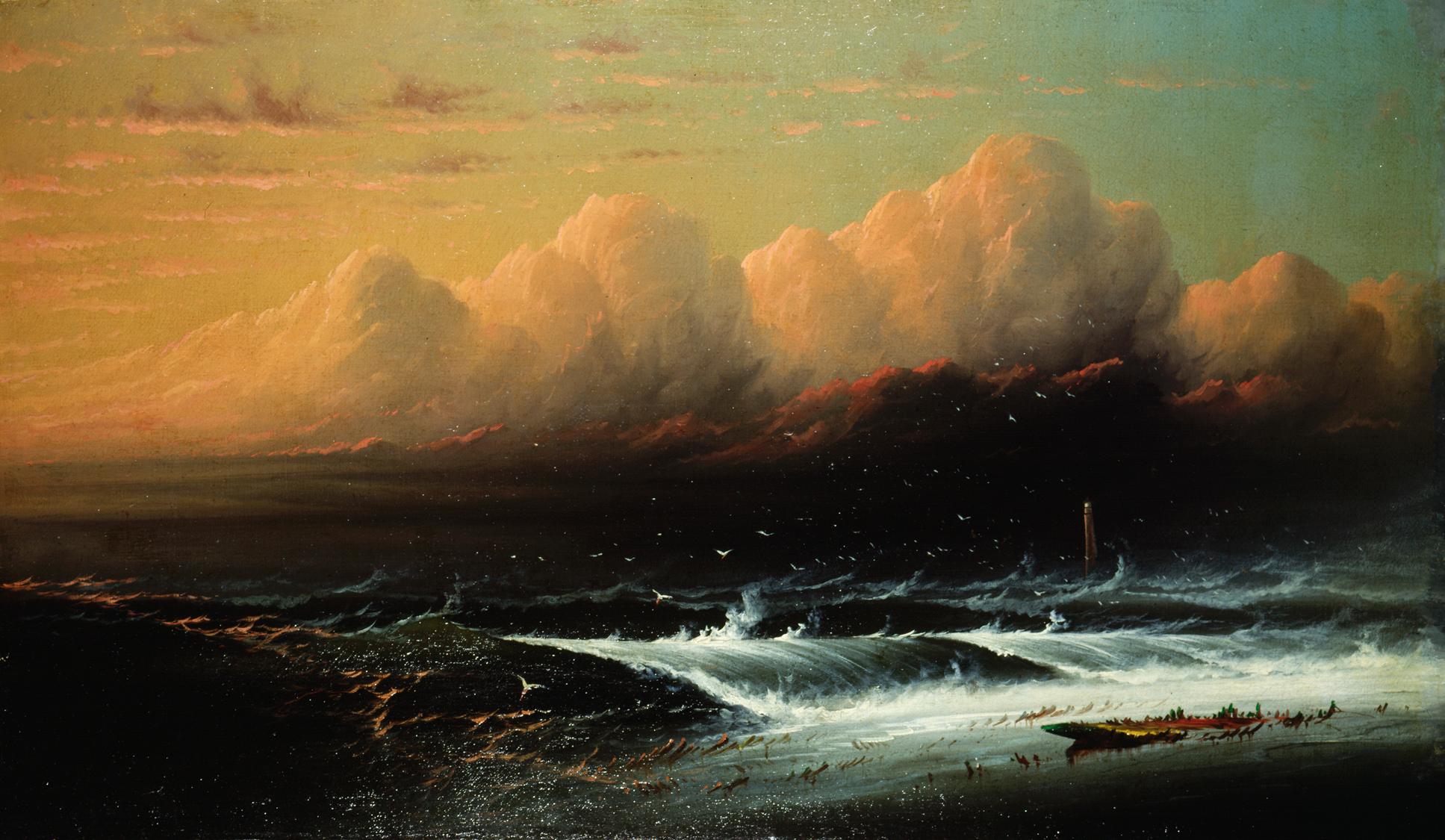This painting depicts a dramatic seascape at sunset, characterized by its bold and contrasting elements. At the very top, the sky transitions from a yellow-green on the left to a more teal aquamarine on the right. Fluffy white clouds tinged with gray sit above darker, more ominous clouds with brown and red hues, suggesting an approaching storm. The horizon features a range of sharp, white-topped clouds that become dark and foreboding toward their base. 

Beneath this striking sky, the ocean dominates the middle and lower portions of the image. The water appears almost pitch black, with tall, formidable waves that crash onto a narrow, dark gray, almost black sandy beach. White birds are scattered throughout the scene, soaring above the waves and landing in the shallow water to the lower left. On the beach at the lower right, there is what seems to be a wrecked wooden boat with grass poking through. Nearby, a colorful rainbow surfboard lies on the sand beside a partially obscured pole or buoy.

Overall, this rectangular painting, roughly three inches tall and six inches wide, captures the raw and tumultuous beauty of the seascape during an intense and vivid sunset, blending vibrant colors with natural chaos.